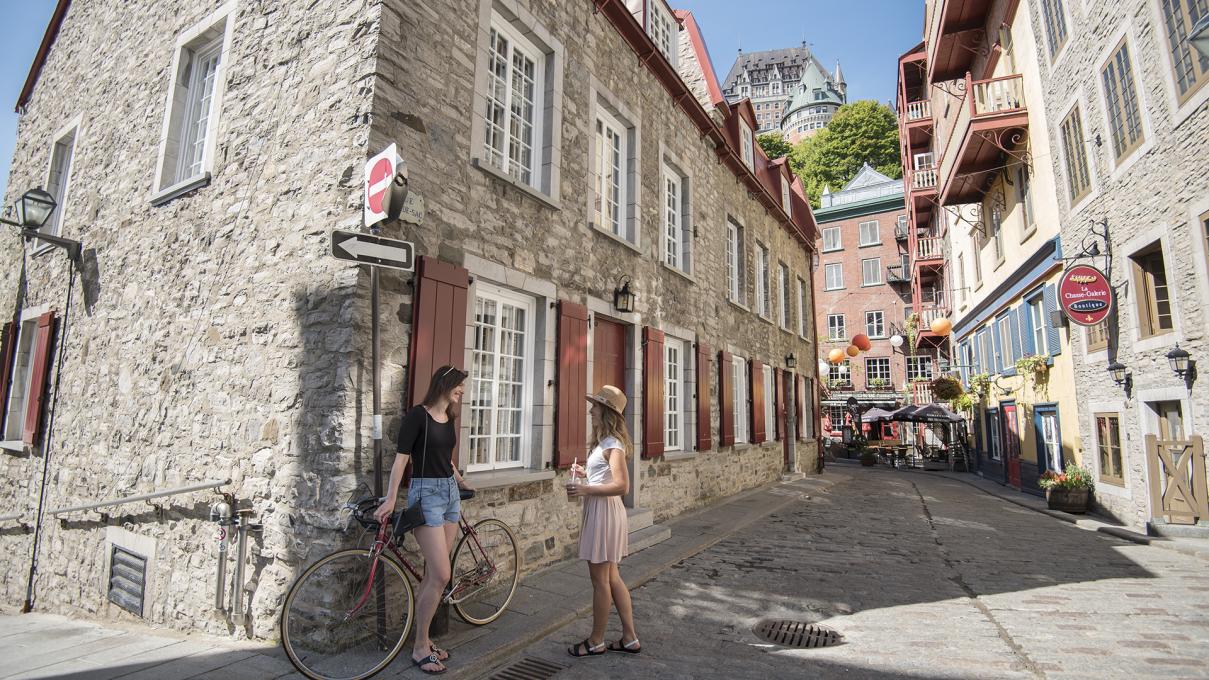In this sunlit photograph, taken in an old-style town with stone streets and narrow sidewalks, two women are engaged in a cheerful conversation on the center-left side of the image. The bright blue sky above casts sharp shadows on the stone buildings, one of which features a row of brown shutters. The taller woman on the left, with long dark brown hair, is clad in a black scoop neck short-sleeved shirt, short denim shorts, and black thong sandals. She leans casually against her bike, which is propped against the wall of the building behind her. Beside her, the shorter woman, wearing a tan hat, a white short-sleeved shirt, and a pale pink skirt that reaches just above her knees, holds a drink as they chat. This woman has blondish brown hair and is smiling warmly. A small stairway ascends into the corner of the scene, while in the background, a pavilion with balloons seems to offer goods for sale. A red circular sign is perched on the upper right, although the text is unreadable. The detailed windows of the buildings and the hints of distant stores and tables add layers of depth to this picturesque street scene.